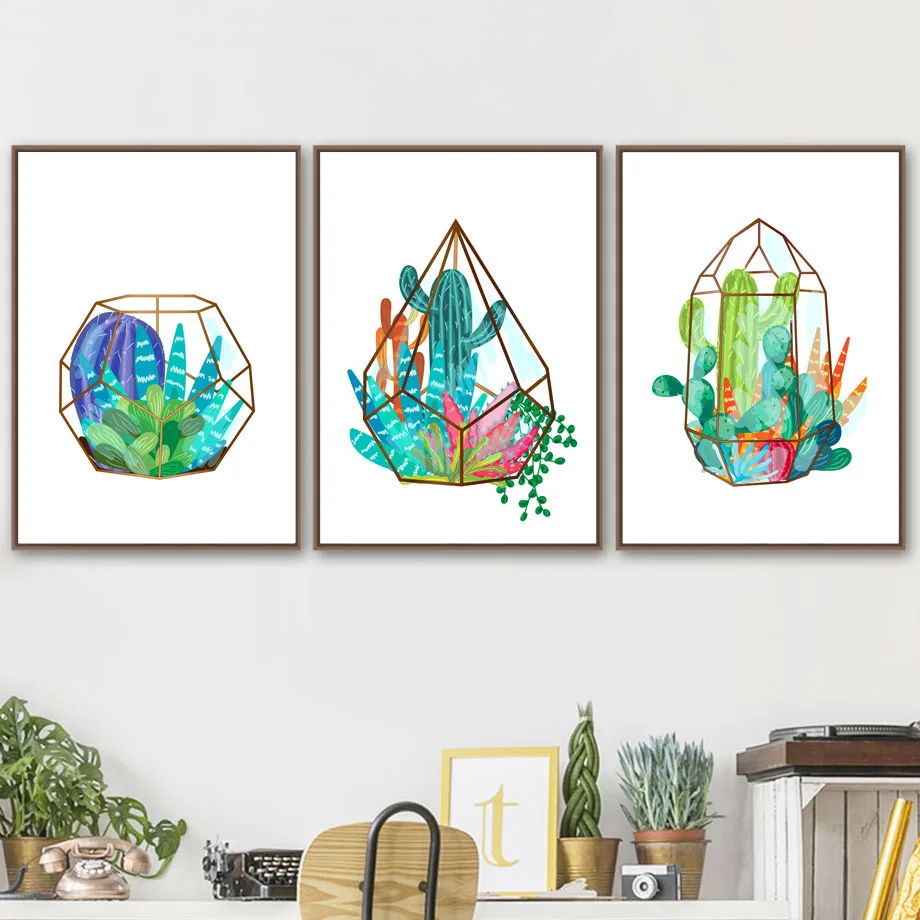The image depicts a neatly arranged home office setup against a bright, white wall. Prominently displayed above a wooden desk are three vertical rectangular picture frames, each the same size and featuring different geometric shapes outlined in gold. The left frame showcases a sphere-like shape with a colorful image of various cacti and plants. The middle frame contains an upside-down diamond shape filled with another variety of vibrant cactus plants. The right frame has a bulkier, wide diamond-like shape, also housing a vivid display of cacti. The color palette of these images includes blues, greens, pinks, purples, and oranges, making the artwork visually striking.

Beneath these frames sits a functional and stylish desk. Positioned on the desk is a gold rotary phone in front of a plant in a gold pot. Adjacent to this is a vintage black typewriter with white keys. You can also spot the back of a wooden chair partly visible. Additionally, the desk holds a small bright gold picture frame with the letter "T" in it, two more gold pots containing green plants, a small camera, and other miscellaneous items. The overall setting is well-lit and clear, providing a welcoming workspace ambiance.